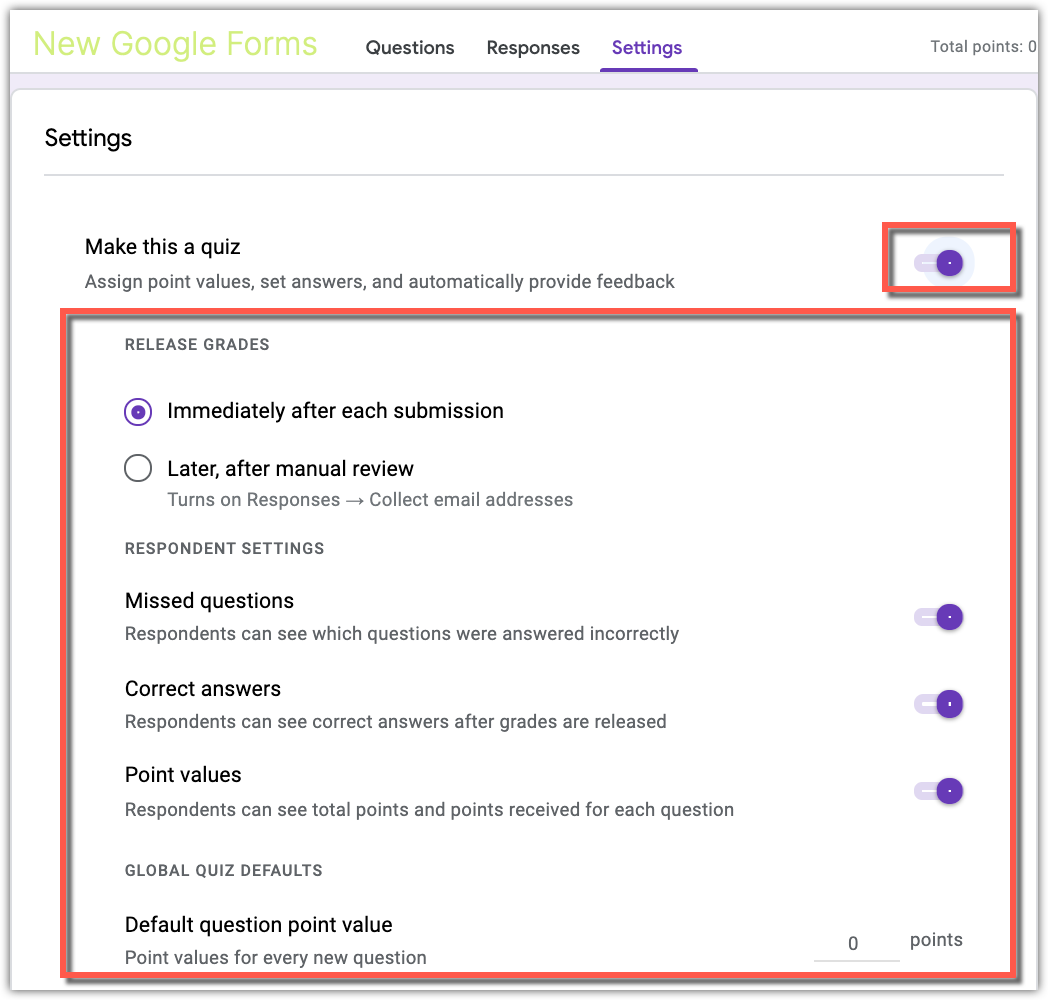In this detailed screenshot, we observe the interface of the new Google Forms set against a white background. The header in the upper left corner features the text "New Google Forms" in yellow. To its right, there are three navigation tabs: "Questions," "Responses," and a purple-highlighted "Settings." 

Within the "Settings" section, several features are outlined and configured. A prominent toggle switch, outlined in red and turned on, allows the form creator to make this a quiz, assign point values, set correct answers, and automatically provide feedback. 

Further down, under the "Release Grades" subheading, there are two options: "Immediately after each submission," which is checked, and "Later, after manual review," which allows for delaying the release of grades. The form setup also includes switches for "Collect email addresses," ensuring respondents' contact information is gathered.

In the "Respondent Settings" section, various toggles manage the feedback visibility:
- "Missed Questions": This toggle is turned on, permitting respondents to see which questions they answered incorrectly.
- "Correct Answers": This is also enabled, allowing respondents to view the correct answers post-grade release.
- "Point Values": Enabled for respondents to see their total points, as well as the points they received for each individual question.

This screenshot exemplifies the detailed and customizable settings available in the new Google Forms quiz feature, enhancing the assessment and feedback process for both form creators and respondents.